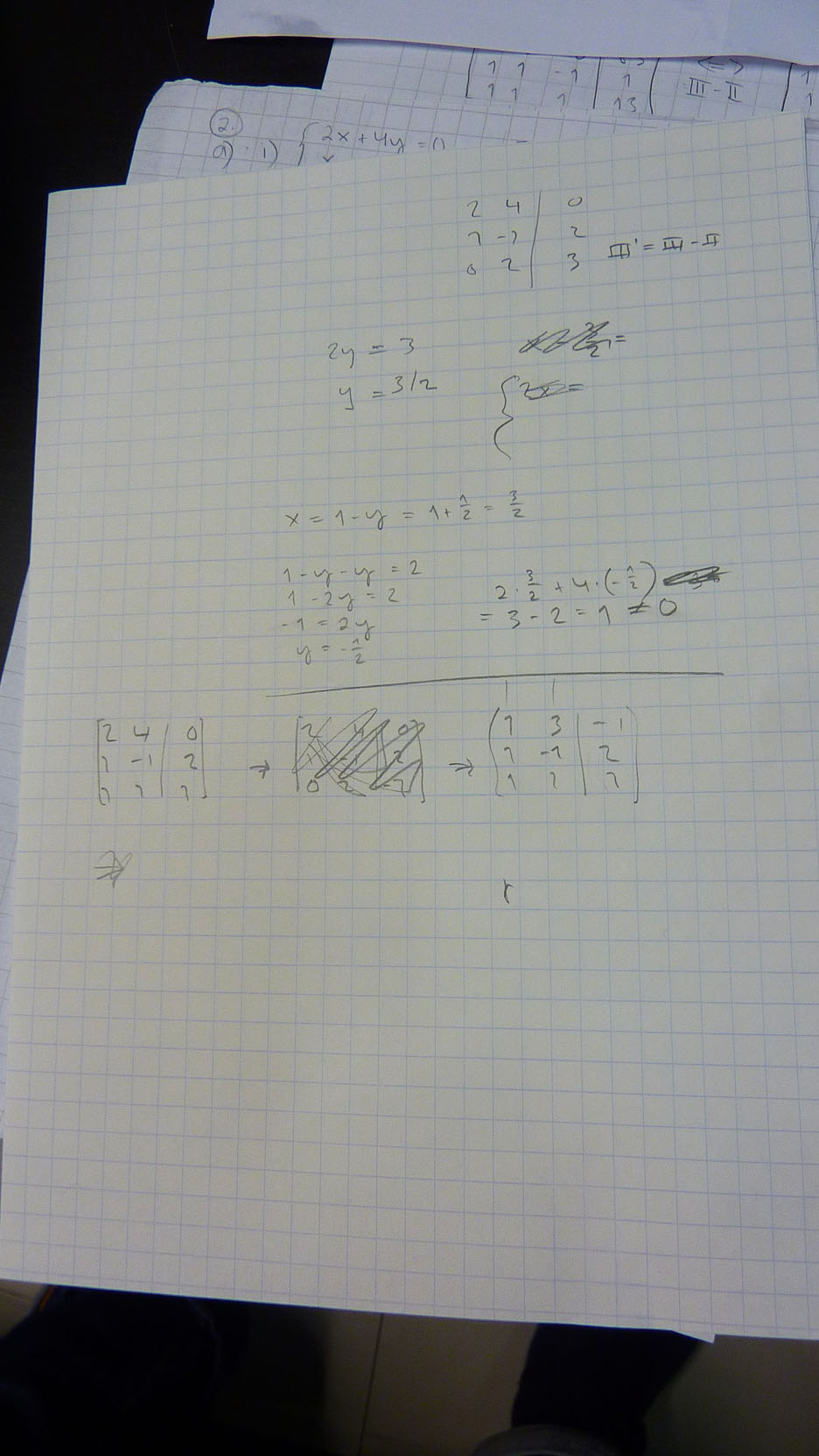The image displays a grid of paper against a mostly black background, filled with handwritten mathematical equations and scratched-out work. The scene seems to depict problem-solving steps for algebraic equations, particularly solving for X and Y.

At the very top, a square on the grid lists the numbers:
- First line: 2, 4 on one side of the vertical line; 0 on the other.
- Second line: 7, -1 with 2, 0, and 2 spaced out on the right; followed by a 3.

Further down, there are scribblings and corrections. On the bottom left, equations include:
- "2Y = 3" followed by "Y = 3/2," resembling a reverse 3.
- "X = 1 - Y," then rewritten as "Y = 1.5."
- Below it: "1 - Y - Y = 2" and "1 - 2Y = 2," concluding with "Y = 0.5" or "Y = -0.5."

On the right side of the paper:
- "2 * 3.5 + 4 * -0.5" followed by scratched-out work.
- Another line reads: "3 - 2 = 1," and questioning its equal to 0.

On the bottom left, another square lists:
- 2, 4, followed by 0, 1, -1, 2.
- Various illegible scribbles and corrections are present.

The endmost square shows different numbers:
- 1, 3, followed by space, -1, 1, -2, 2, and another batch of numbers: 1, 2, 2.

The handwriting remains challenging to decipher throughout, and behind this main paper, there are additional sheets filled with formulas, such as "2X + 4 = 0," and more squares with points in them.